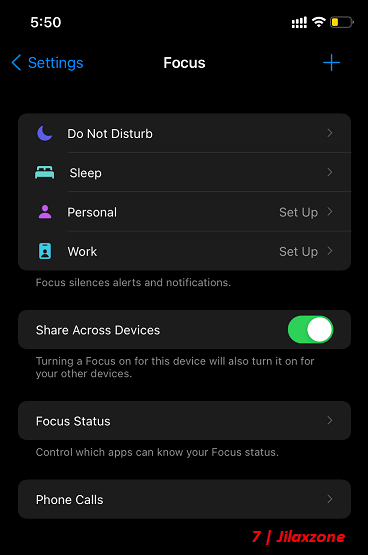The image depicts a smartphone screen displaying the "Focus" settings page in a dark-themed interface, where the primary colors used are blue, green, yellow, purple, and red. 

At the top, the status bar shows indicators for cellular signal, Wi-Fi, and battery level, all represented in yellow. The number '550' appears on the left of the status bar. 

Directly below the status bar, there's a back arrow labeled "Settings" on the left. The title "Focus" is centered in white text, with a blue plus sign on the right.

The main section is divided into several focus modes, each on a slate gray background with white text and a right arrow indicator:

1. **Do Not Disturb**
2. **Sleep**
3. **Personal** - Accompanied by a "Set Up" label on the right.
4. **Work** - With a "Set Up" label on the right.

Below these options, a description reads: "Focus silences alerts and notifications," in small font. 

A toggle bar labeled "Share Across Devices" is activated in green. Underneath this, explanatory text states, "Turning a focus on for this device will also turn it on for your other devices."

Further down, there's another right arrow next to "Focus Status," with smaller text below it explaining, "Control which apps can know your Focus status."

Lastly, "Phone Calls" is listed with a right arrow, and the bottom right corner features a label in red text, "J-I-L-A-X-Z-O-N-E."

The overall background is predominantly black, with the aforementioned sections and settings distinctly highlighted for clarity.